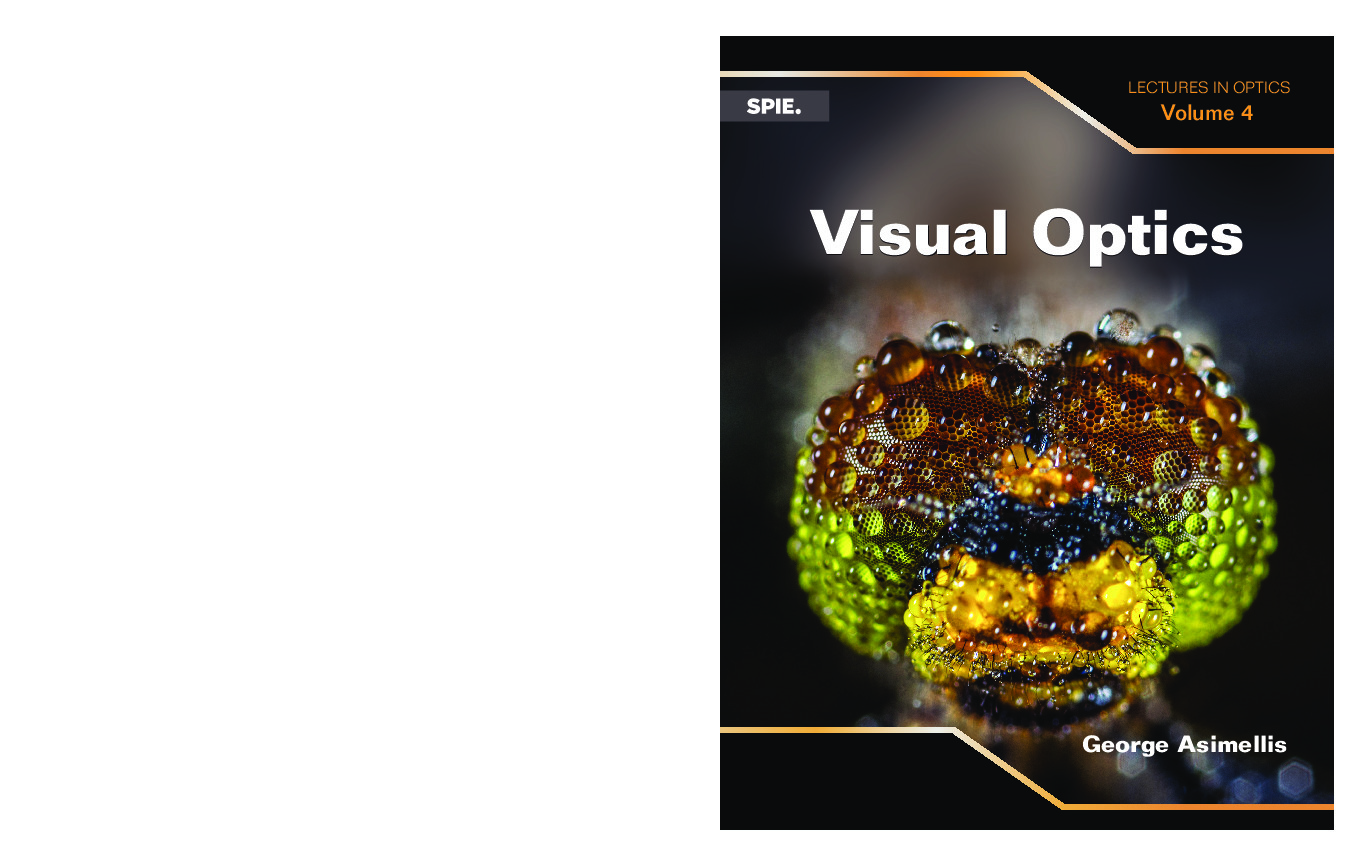This cover of a catalog features a striking design set against a solid black background. In prominent white lettering, "Visual Optics" headlines the cover, while the author's name, George S. Mellis, is displayed at the bottom. Denoted in the upper left is "SPIE," indicating the publisher, and in an orange font in the upper right, it reads "Lectures in Optics, Volume 4." Both the top and bottom of the cover are bordered by an orange gradient line that angles downward, creating a unique step-like pattern. 

Central to the cover is an intriguing glass object, composed of numerous textured, knob-like protrusions that give it a round, multi-faceted appearance. The object displays a rich palette of colors—brown at the top, green on the sides, dark black at the front, and splashes of yellow underneath. This intricate glass form rests on a glass table, casting a partial reflection that adds depth to the image. The detailed textures and vivid colors invite viewers to ponder the object's nature, encouraging a deeper engagement with the visual aesthetics of optics.